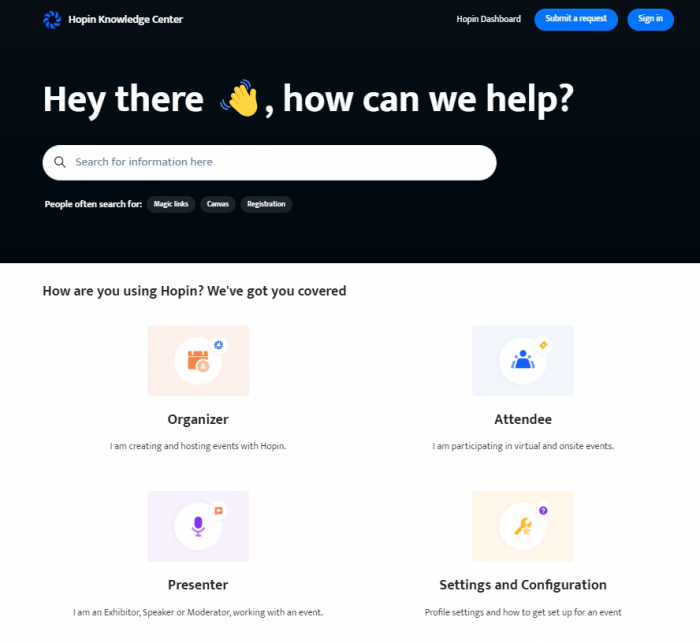The Hopkins Knowledge Center website features a distinctive layout with a flower-like logo composed of blue petals positioned alongside the site name in the top left corner. On the same row on the top right, there is a navigation bar with a "Hop-in Dashboard" label and two blue buttons: "Submit a Request" and "Sign In." 

The header of the website, adorned in black and occupying a significant portion of the page, showcases a greeting in large white text that reads, “Hey there! How can we help?” accompanied by an icon of a hand waving. Below this welcoming message is a search bar, providing easy access to site-wide information, and three quick-access tags: "Magic Links," "Canvas," and "Registration."

Transitioning from the header, the main content area features a white background. The section begins with a title stating, "How are you using Hopin? We've got you covered." This area is divided into four sections, each tailored to a specific user role and identified by a corresponding icon above its title:

1. **Organizer**: Represented by an icon resembling a tower.
2. **Presenter**: Marked by a purple microphone icon.
3. **Attendee**: Illustrated with a blue silhouette of a person.
4. **Settings and Configuration**: Symbolized by a graphic of a wrench and a yellow star.